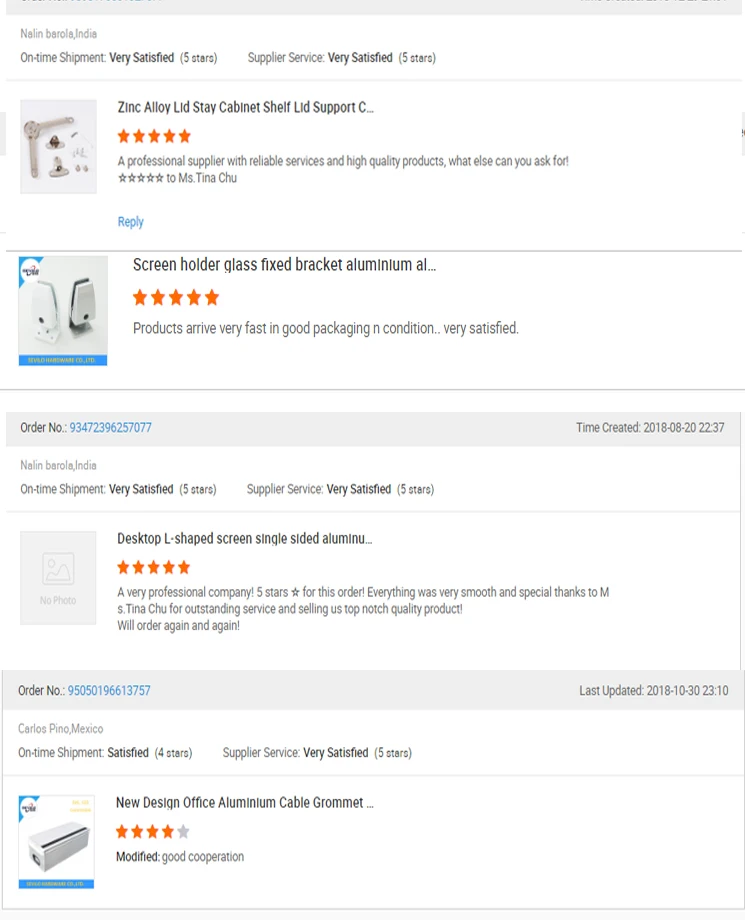This image showcases a detailed review of various items listed on an online store, complete with ratings and descriptions in a foreign language. From top to bottom, here's what it includes:

1. **General Overview**:
    - **One-time shipment**: Rated five stars for customer satisfaction.
    - **Supplier Service**: Also rated five stars, indicating highly reliable service.

2. **Product Descriptions and Ratings**:
    - **Zinc Alloy Shelf Support**:
        - Product description: "Zinc alloy LTD stay cabinet shelf support."
        - Supplier Description: "A professional supplier with reliable services and high-quality products."
        - Customer rating: Five stars for overall satisfaction.

    - **Screen Holder with Glass Fixed Bracket**:
        - Product description: "Glass fixed bracket made of aluminum."
        - Customer feedback: "Product arrived quickly, well-packaged, and in excellent condition."
        - Customer rating: Five stars for overall satisfaction.

    - **L-shaped Desktop Screen Holder**:
        - Product description: "Single-sided aluminum L-shaped screen holder."
        - Customer ratings: Five stars for the product and the professional company fulfilling the order.
        - Customer feedback: "Everything was smooth."

    - **New Design Aluminum Cable Grommets**:
        - Product description: "New design, alumina cable grommets."

3. **Additional Details**:
    - **Order Number**: Displayed at the bottom of the image.
    - **Shipment Details**: One-time shipment noted multiple times.

This review image highlights customer satisfaction with high quality and reliable products, indicating a trustworthy and efficient supplier.